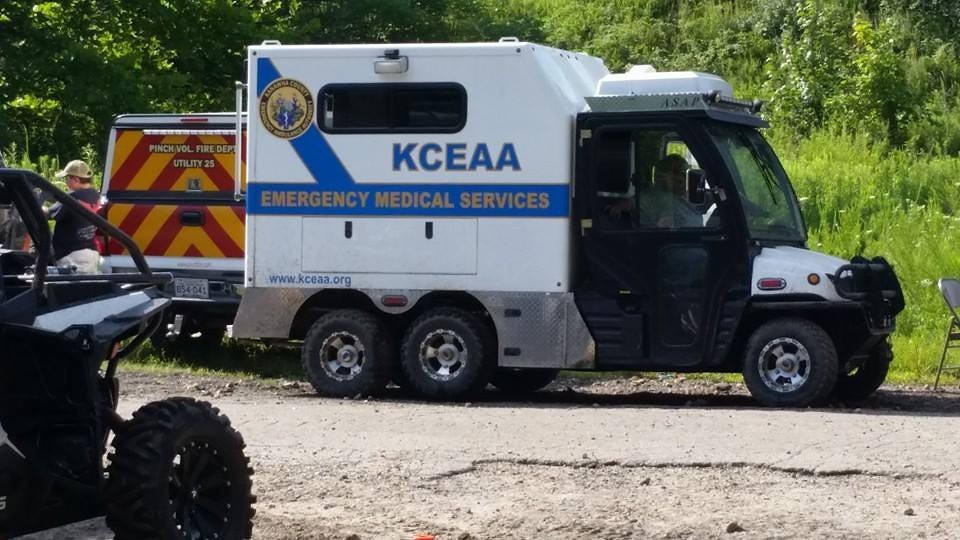The photograph captures a bustling emergency scene set in a rural, forested area. Dominating the center of the frame is a white and blue medical vehicle with "KCEAA" emblazoned in large blue letters and "Emergency Medical Services" written in gold below a diagonal blue stripe. This vehicle, possibly an ambulance, has a white back with a rectangular window and a blue banner along its side. In the foreground, at the lower left corner, a dirt bike is partly visible with a woman standing behind it. Directly behind the ambulance is a red and yellow striped utility truck from the "Pinch Volunteer Fire Department," labeled "Utility 25," hinting at its role as a paramedic fire department vehicle. To the right of this utility truck, partially obscured, is a man wearing a cap. The scene is set on a rutted dirt road, with tall grass and trees forming the backdrop, emphasizing the rural, off-road setting.